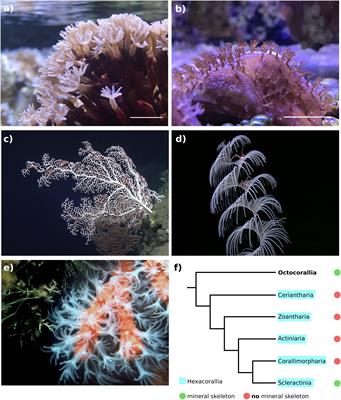The image is a detailed photograph broken into four quadrants and labeled from A to F. Each section showcases different coral species commonly found in the ocean. 

- Section A presents a light brown, cylindrical coral with delicate, white strands extending from its tip, resembling upside-down squid tentacles.
- Section B features a similar coral structure, but in shades of pink, with more foliage visible in the background.
- Section C depicts a coral that appears at night, lit in black and white, showing a white vein with darker, web-like extremities.
- Section D resembles a drawing under a black background, displaying layers of white, thin, strand-like leaves hanging down like a weeping willow.
- Section E shows coral with an orange vein and white-green flowers, resembling dandelion wisps, set against a darker backdrop with some foliage.
- Section F is a chart detailing the coral classification, featuring an unreadable legend with various colored balls connected by lines. The labels include "octocorallia," "choriantharia," "zoantheria," "actinaria," "chorallimorpharia," and "selenoconia," with associated symbols for "mineral skeleton" and "no mineral skeleton."

This highly detailed image underscores the intricate features and classification of various coral species, highlighting their unique visual characteristics.